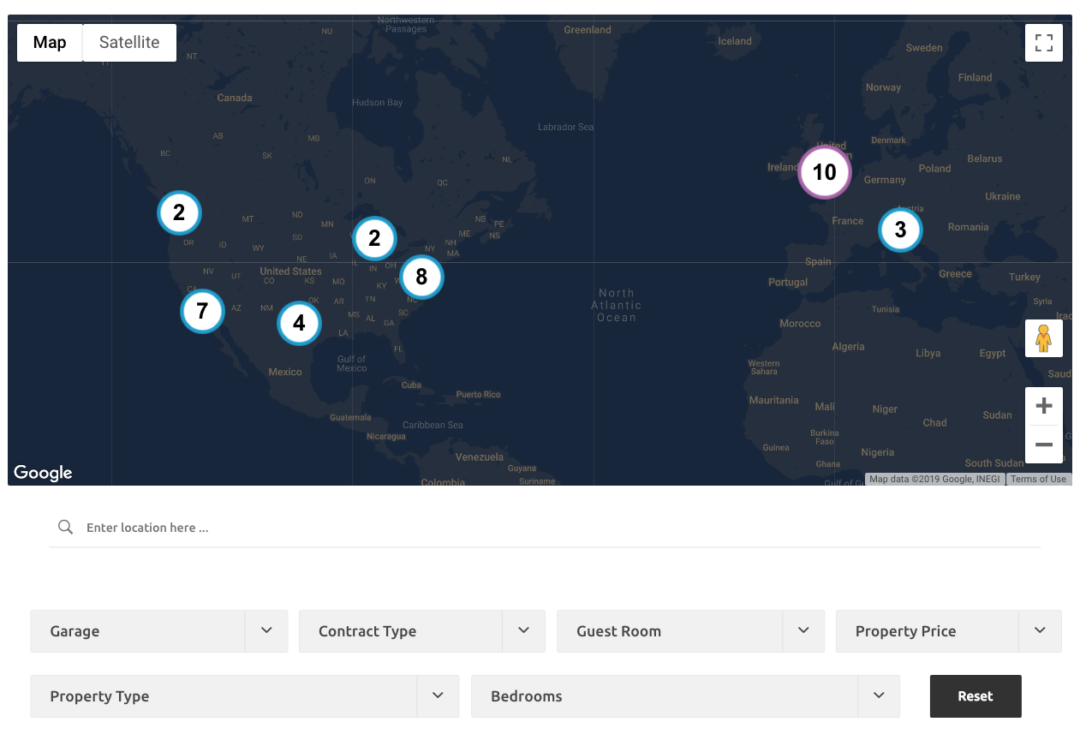The image depicts a digital interface for a real estate application, featuring a world map with a satellite view. The map is primarily blue, with continents outlined in a teal-green color. Various numbers, including "2", "2", "7", "4", "8", "3", and "10", are displayed on the map, presumably indicating data points or locations, though their specific significance is unclear.

Below the map, there are input fields labeled "Enter location here," suggesting that users can enter a specific location to search for. Additional sections include dropdown menus for "Garage," "Contract Type," "Guest Room," "Property Price," "Property Type," and "Bedrooms," each allowing for user customization in their search criteria. These dropdown menus are gray with white text, except for the last one which features a black background with white lettering.

A "Reset" button is also present, enabling users to clear their selections and start a new search. The numbers on the map are distributed across various regions, with most concentrated in the United States and only a few in other countries. The interface overall appears to be a real estate search tool, though further context or instructions are not provided in the image.